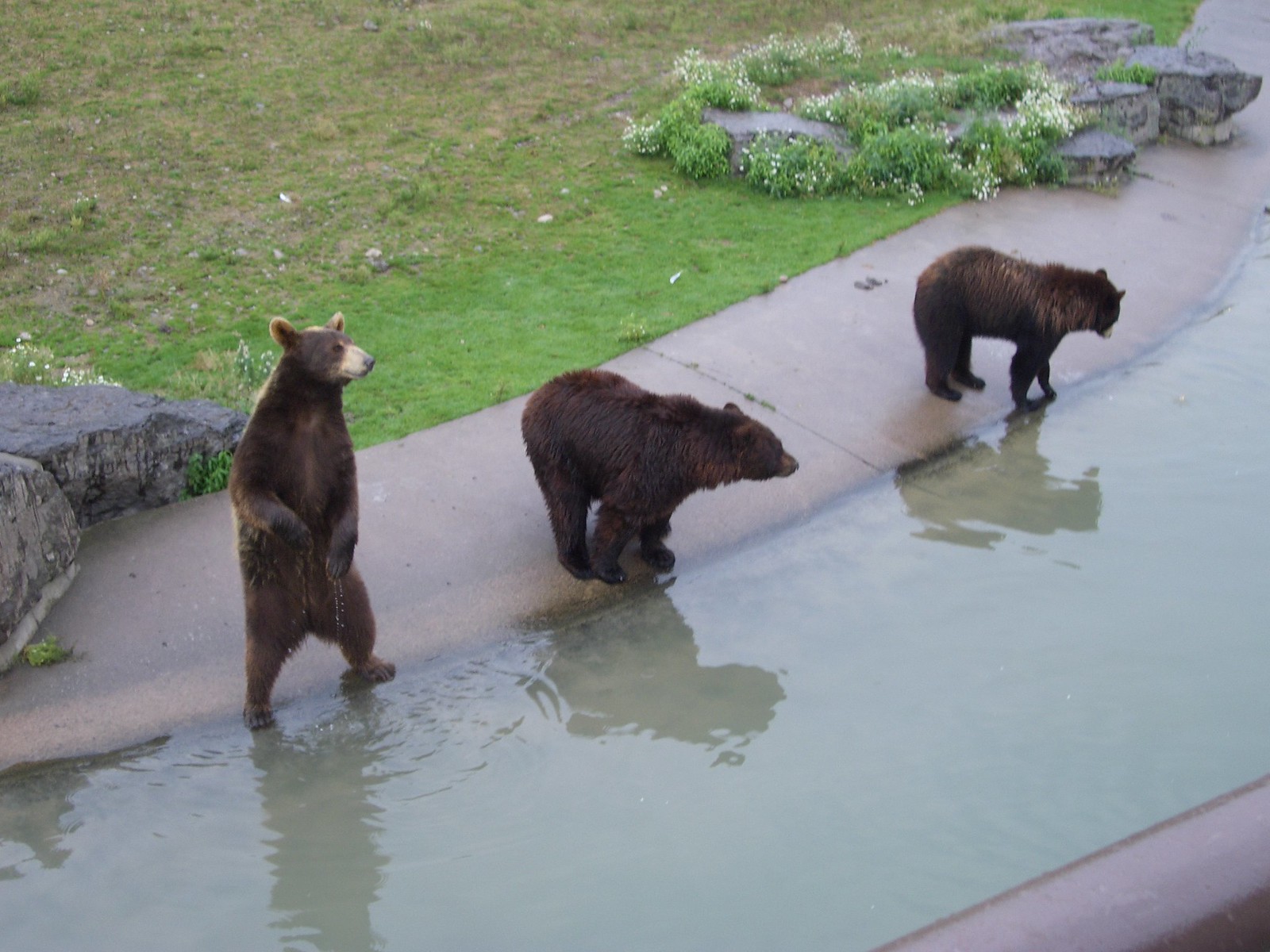This vibrant photograph captures a scenic zoo enclosure featuring three dark brown bears at a water-filled moat. The bears, likely black bears given their dark hue, are positioned along a rectangular concrete waterway which spans the foreground of the image and continues along the right edge. The water in the moat is clear blue, mirroring the reflections of the bears. 

The bear on the left stands erect on its hind legs, gazing intently to the right, while the middle bear crouches on all fours, looking slightly to the left. The bear on the far right, which appears to be smaller, remains on all fours with its head bowed downwards. Behind these majestic creatures lies a lush green lawn dotted with white wildflowers and various low-lying plants, bordered by large gray boulders on both sides. The scene, part of a well-designed zoo habitat, is both naturalistic and secure, ensuring the bears have ample space to roam while keeping them safely separated from visitors admiring them from a distance.